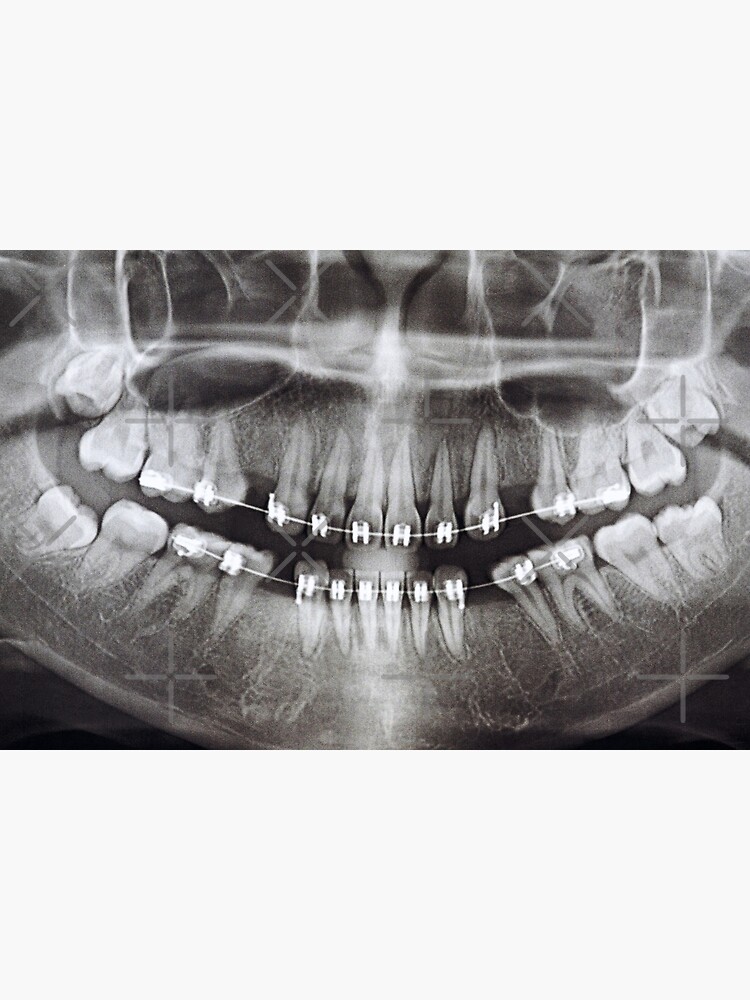The image depicts a professionally taken, black-and-white x-ray of an adolescent's lower face, focusing primarily on the mouth and teeth. The top third of the image is a plain white background, while the bottom two-thirds showcase the x-ray details. At the top of the x-ray, just the tip of the nose is visible, followed by the oval shape of the mouth with lips slightly parted into a smile. The grin reveals the top and bottom rows of teeth, with teeth in the center clearly visible and side teeth curving around the jaw. A notable feature on the bottom left is a partially erupted molar, likely a wisdom tooth, still mostly below the gum line.

The teeth appear in shades of gray, while the metal braces they are wearing stand out in bright white. These braces consist of small H-shaped brackets affixed to each tooth, connected by a wire threading through each bracket. There are approximately 8 brackets on both the top and bottom rows of the teeth, and each wire is secured by clasps at the ends. Additionally, parts of the nasal cavity are faintly visible, but the main focus remains on the teeth and orthodontic apparatus, suggesting the image could serve educational purposes, possibly illustrating proper dental alignment for students or patients.